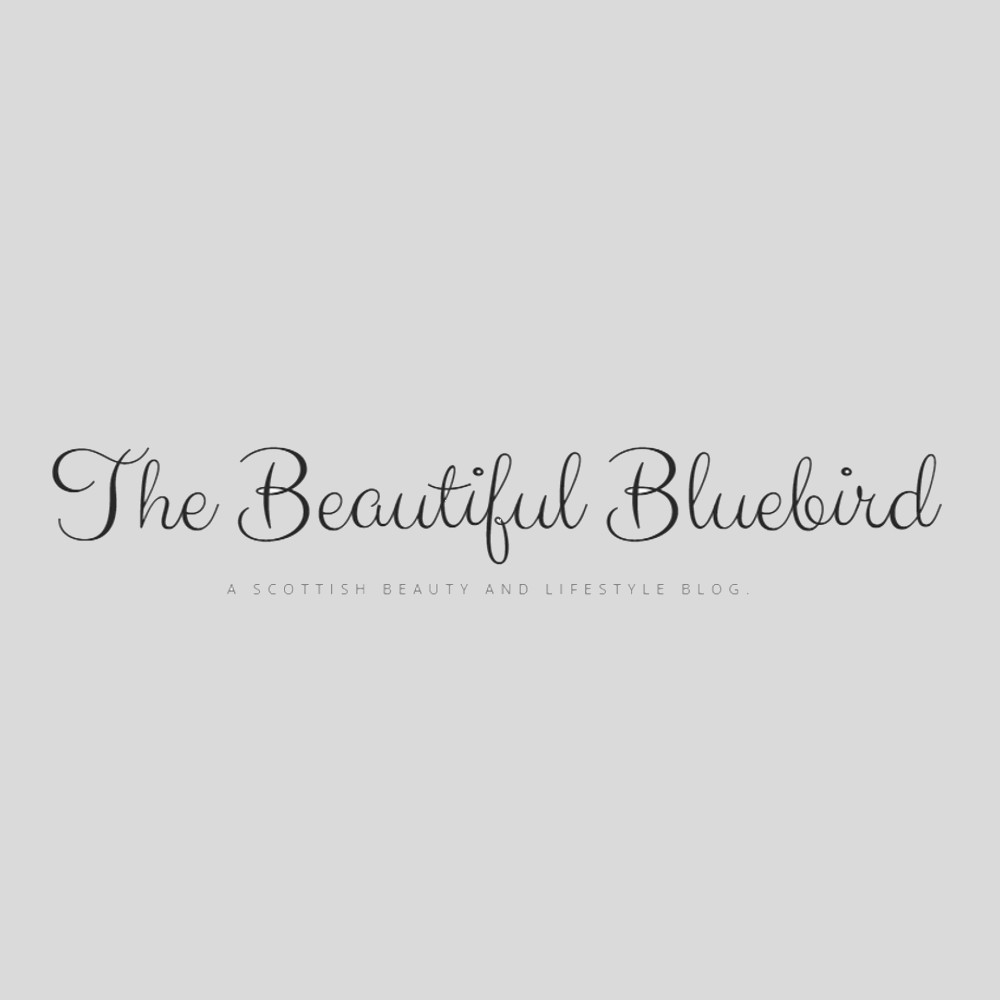The image features a nearly square design with a light gray background. Prominently displayed in the center is the text "The Beautiful Bluebird" in a stylish, dark cursive font that lends a dainty and elegant appearance. Below this, in all capital letters and a smaller, more straightforward font such as Arial or Roman, the text reads "A SCOTTISH BEAUTY AND LIFESTYLE BLOG." The contrast between the elaborate, connected cursive and the clean, spaced-out capital letters below is particularly striking, lending the image a professional and polished look.